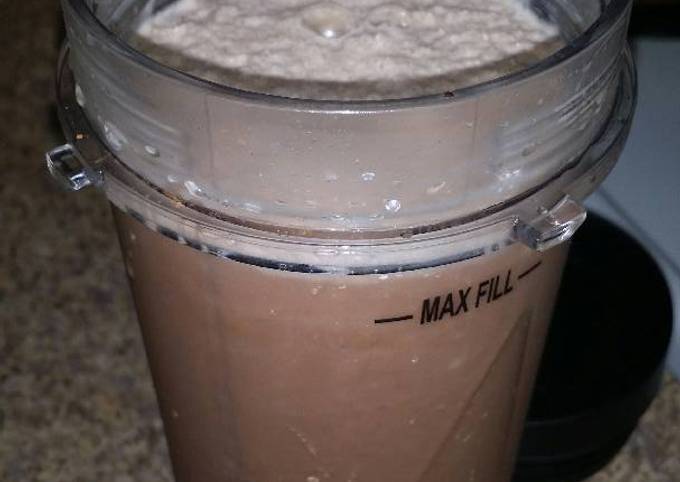In the image, a clear plastic blender cup prominently sits on a light-colored granite countertop adorned with gold and brown flecks. The lid of the blender cup is unscrewed and positioned next to it on the counter. The blender cup, almost filled to its brim and exceeding the "max fill" line indicated by black lettering, contains a brown, chocolate-flavored milkshake with a half-inch layer of creamy, off-white foam and bubbles on top. The exterior of the cup shows signs of condensation, with droplets streaming down its side. The detailed granite countertop highlights the blender cup as the central focus amidst the earthy tones of the background.